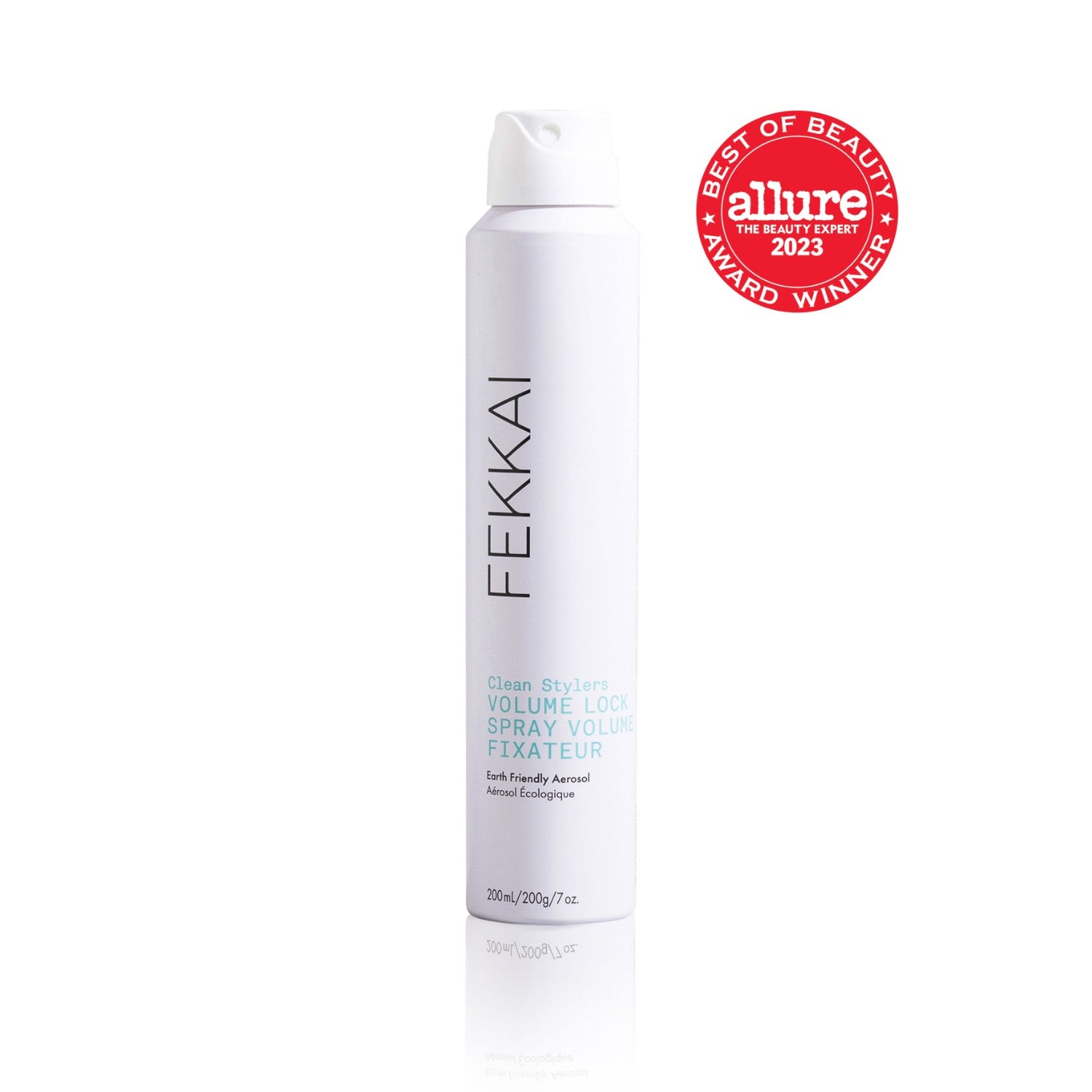The image serves as an advertisement for a beauty product. It features a white spray bottle prominently labeled "FEKKAÏ" in bold black letters. Below, in aqua lettering, it includes the text “Clean Stylers, Volume Lock Spray, Volume Fixature.” Further down, in smaller black text, it states, “Earth Friendly Aerosol / Aerosol Écologique.” The bottom of the bottle lists its size as "200 ml / 200 G / 7 OZ." The bottle is designed with a round, short sprayer reminiscent of foaming sunscreen sprays. This product’s photograph is set against a plain white background, with the bottle's reflection visible on the white surface. On the top right of the image, a red circular label declares the product as an "Allure 2023 Best of Beauty Award Winner" with the words "Allure The Beauty Expert" in white lettering.